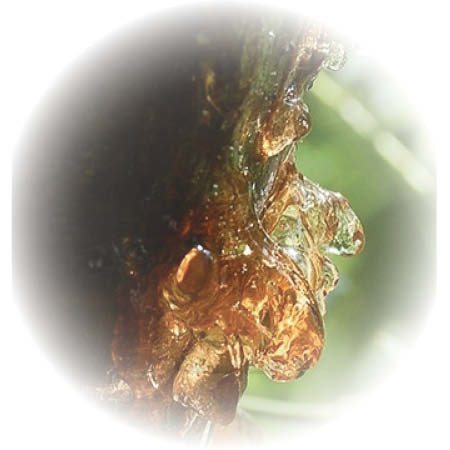The image presents a blurred circular frame with no border, placed on a white background. The focal point within the circle reveals what appears to be a detailed, side view of a wooden or metal statue of a man's face. This statue, which might also be interpreted as hardened tree sap, exhibits a flat forehead leading into the curve down the left side forming the back of the head. The face of the figure shows a pronounced long, pointy nose, an outlined eye, the curve of the mouth, and down to the chin, which then transitions into the neck. The material reflects a mix of brown, gold, and green hues, giving it an amber-like appearance with some parts clear and jelly-like. The upper and lower regions are hazy, enhancing the sense of depth and the play of light on the shiny surface. The background is an out-of-focus combination of light and dark green shades, suggesting foliage or leaves, and it appears bright as light filters through.